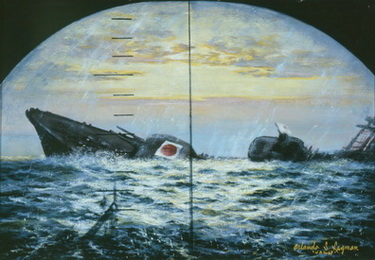In the painting, we see a dramatic naval scene viewed through a submarine's periscope, indicated by the rounded top and vertical notches framing the circular image. The setting sun or rising sun bathes the sky in a yellowish-red hue, blending with light blue and orange shades. The ocean below is rough with choppy waves, creating a tense atmosphere. In the distance, a battleship with a Japanese flag is severely listed, sinking with both ends of the ship raised out of the water, and a gun turret bearing the flag is prominently featured. Another freighter to the right appears on the verge of capsizing. The entire scene, although artistically muted with a mix of black and white tones interspersed with color, vividly captures the moment of destruction. The artist's signature is subtly present on the bottom right of the rendering.